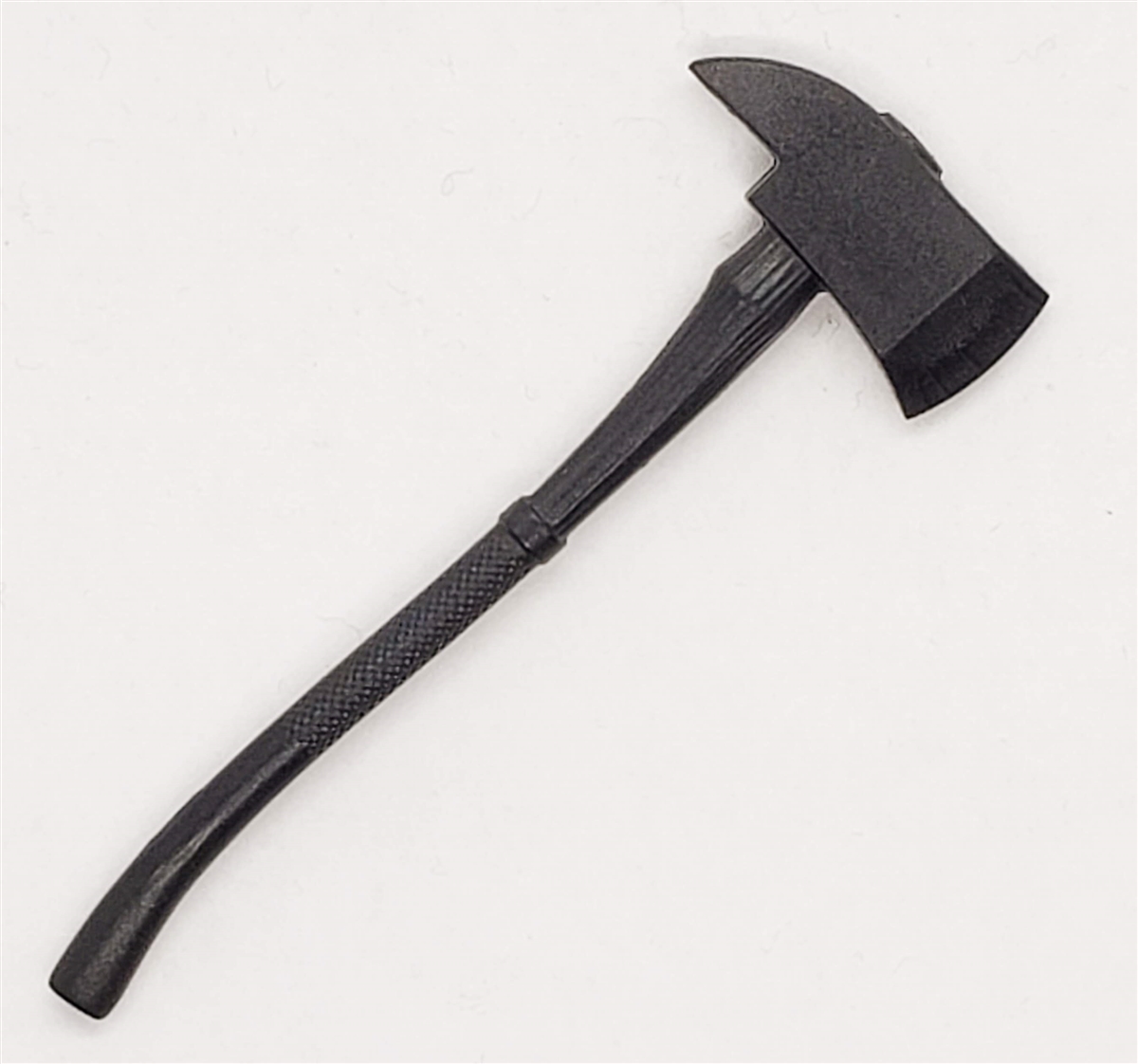This detailed photograph showcases a modern, non-traditional small axe set against a white background. The axe features an almost uniformly dark grey, nearly black color. Its long, thin handle includes a patterned, raised grip area, designed to enhance friction and improve handling. The axe head includes a distinctive sharp edge at the front, which is jet black, and curves in a bow-like shape. The back of the axe head tapers to a stubby yet powerful section suitable for chopping. The overall design suggests it may not be intended for heavy-duty wood chopping but is more likely suitable for lighter tasks like preparing campfires. The design and color suggest that it could even be a modern or 3D-printed prop.